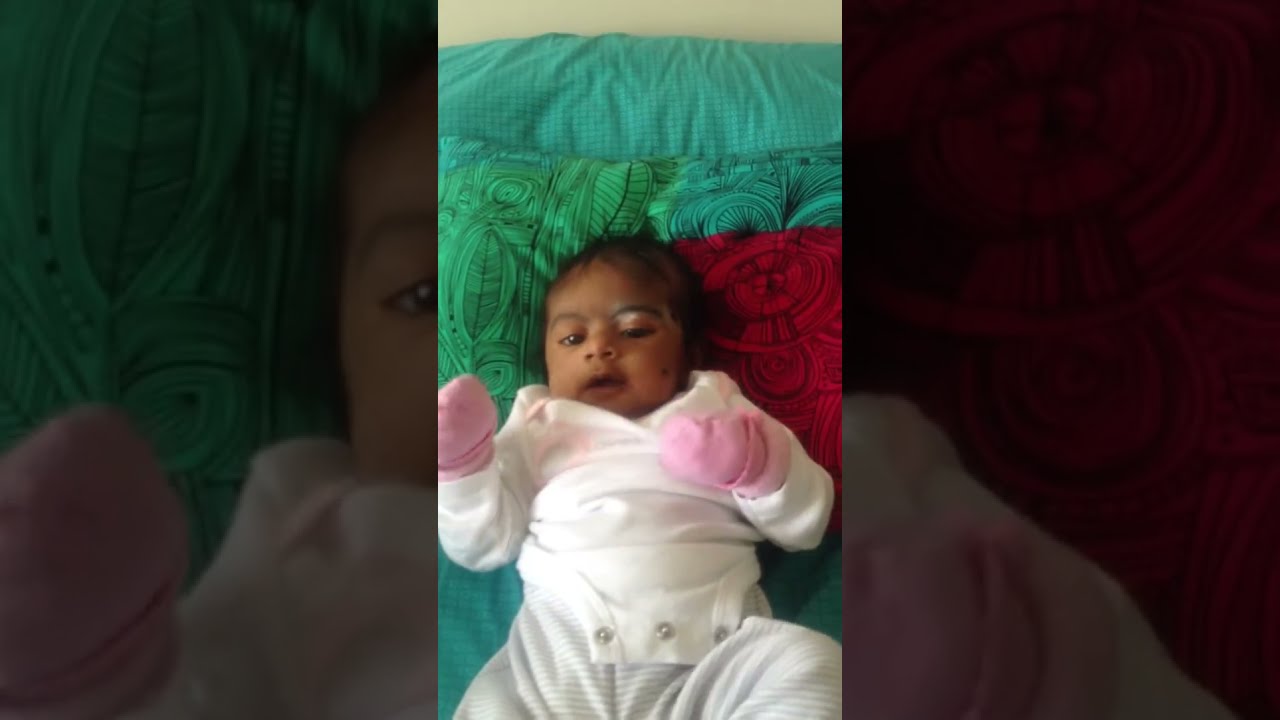This image showcases a very young infant, lying on their back on a bed or cushioned area. The background features green fabric, supplemented with a red pillow and additional brown and possibly blue pillows. The baby, who appears to be a few months old and of Indian descent, has a dark complexion, with black or dark brown hair. Their eyes are open wide, giving a stern or serious expression as they look toward the lower right side of the image. The infant is dressed in a white onesie that remains unbuttoned at the bottom, likely for easy diaper changes, and is paired with white and light blue striped pants. To prevent scratching or getting tangled in their hair, the baby's hands are covered with pink mittens.